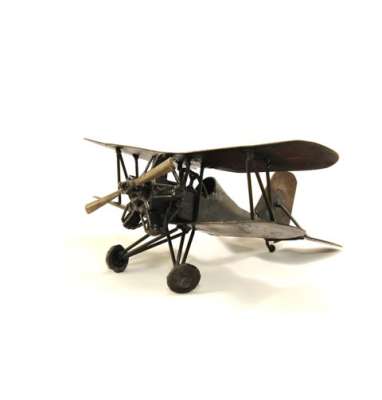The image showcases a detailed model of an old-fashioned biplane, predominantly made of bronze metal that exhibits a rustic color reminiscent of early aviation history. The airplane, resembling early models designed for one or two passengers, features a large wing on top and another on each side of its fuselage. A single two-blade propeller is mounted at the front of the biplane, which rests on two front wheels and one smaller rear wheel, positioned slightly off-center to the left on the white background. The tailplane, standing upright, casts a distinguished shadow on the surface below, contributing to the photo's nostalgic ambiance. This metallic biplane model, with its intricate details, evokes the pioneering spirit of early aviation.